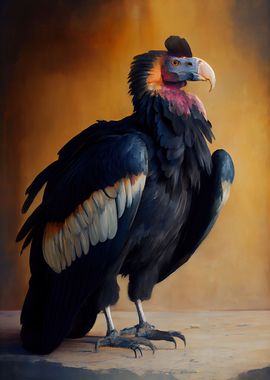The photograph captures a majestic, massive bird that exudes a sense of grandeur and no-nonsense demeanor. Dominating the composition, the bird's imposing presence is highlighted by its predominantly black plumage, which covers its face, chest, and most of its body. A striking contrast is provided by the bird’s beak, which is a pale peach or beige hue, and its neck, adorned with a mosaic of magenta, purple, and black feathers that add a vibrant splash of color.

The bird's wings are a complex tapestry of navy blue, orange, white, and black feathers, with a distinctive diagonal white patch patterned with orange. Its legs are a sturdy gray, ending in dark gray feet equipped with sharp talons, suggesting both strength and agility. The bird stands firm on a somewhat peachy-gray stone platform, which appears weathered and slightly patchy.

The background of the image is predominantly orange, suffused with golden light that seems to emanate around the bird, enhancing its regal appearance. Dark brown hues accentuate the top corners, especially on the left, fading gradually toward the center, and more quickly on the right side. This dramatic backdrop not only frames the bird but also emphasizes its commanding presence, elevating the overall aesthetic of the photograph.